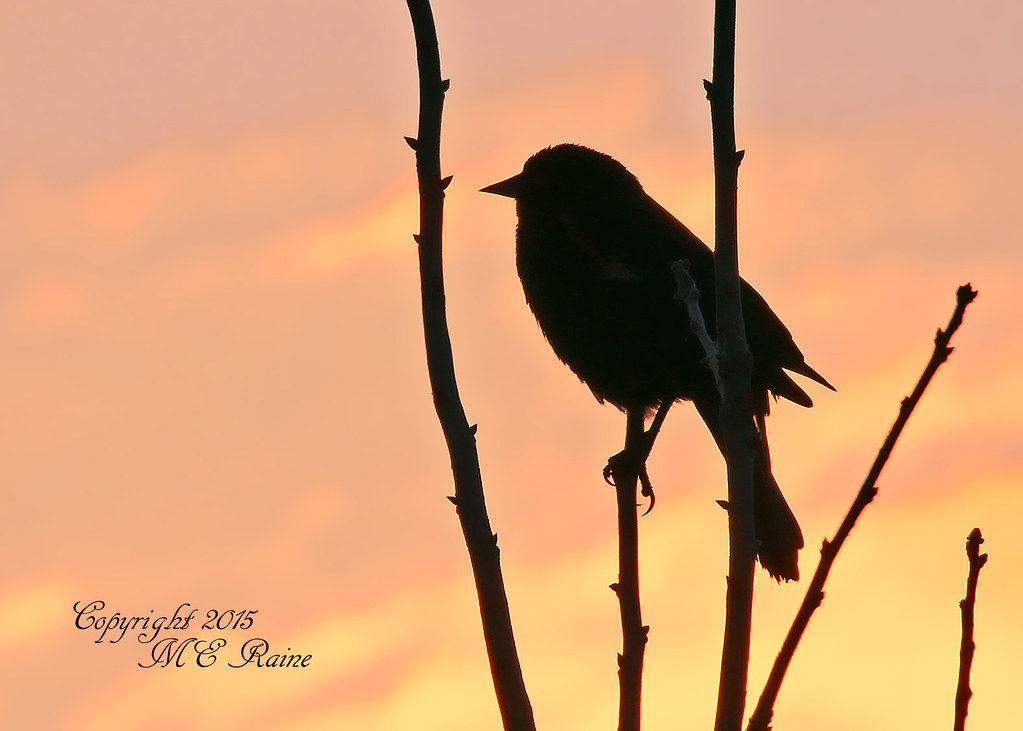This captivating photograph features a silhouetted bird perched on one of five visible branches, all devoid of leaves and buds beginning to form. The bird is positioned in profile, with its sharp, short beak facing left and its tail to the right, gracefully sitting on the second branch from the bottom. The vibrant sky transitions from a deep orange with hints of yellow in the top left to a more yellowish hue towards the bottom right, creating a beautifully contrasting backdrop. At the lower left corner of the image, delicate cursive text reads "copyright 2015 M.E. Rain," marking the artist's signature. The scene exudes a tranquil, twilight ambiance, perfectly capturing the serene moment of a bird at sunset.